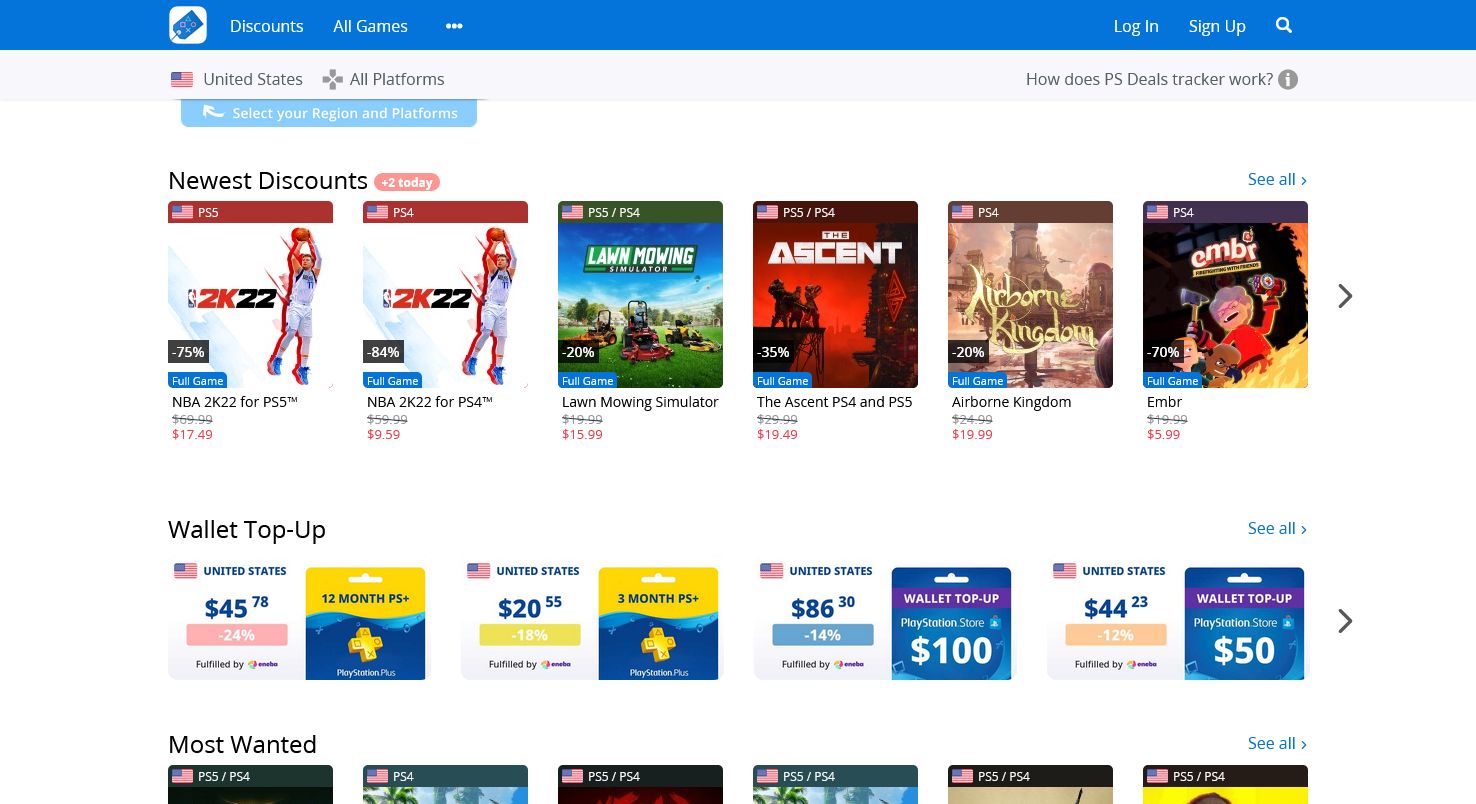The image displays a detailed screenshot of a shopping website dedicated to video game discounts. At the top, there is a medium blue header featuring a white square icon with a blue price tag and video game controls, accompanied by the text "Discounts" in white letters. To the right of this, the menu options "All Games" and a set of three dots are visible. 

On the far right, in the same blue header, the options "Login" and "Sign Up" are displayed in white letters, alongside a white magnifying glass icon indicating a search function. 

Below the blue header, on the left, an area displays the United States flag with the text "United States" next to it. To the right, there is a plus sign and the text "All Platforms". Further to the right, under the blue header, the text "How does PS Deals Tracker work?" appears in medium gray letters, accompanied by a dark gray circle containing a white letter 'i'.

Beneath the United States and "All Platforms" section, there is a light blue bar with a white upward-swooping arrow pointing towards the flag, and to its right, the text "Select your region and platforms". 

The main content area is divided into sections. The "Newest Discounts" section lists six PS4 games. Adjacent to "Newest Discounts," the text "Plus 2 Today" is highlighted in red. Below this, the "Wallet Top-Up" section displays various top-up options, eight in total, represented by little squares. One of these options for the United States is a white square labeled "$45.78" with a red bar below indicating "Minus 24%".

Further down, the "Most Wanted" section lists six video games available for both PS5 and PS4, specifically showing deals applicable to users in the United States.